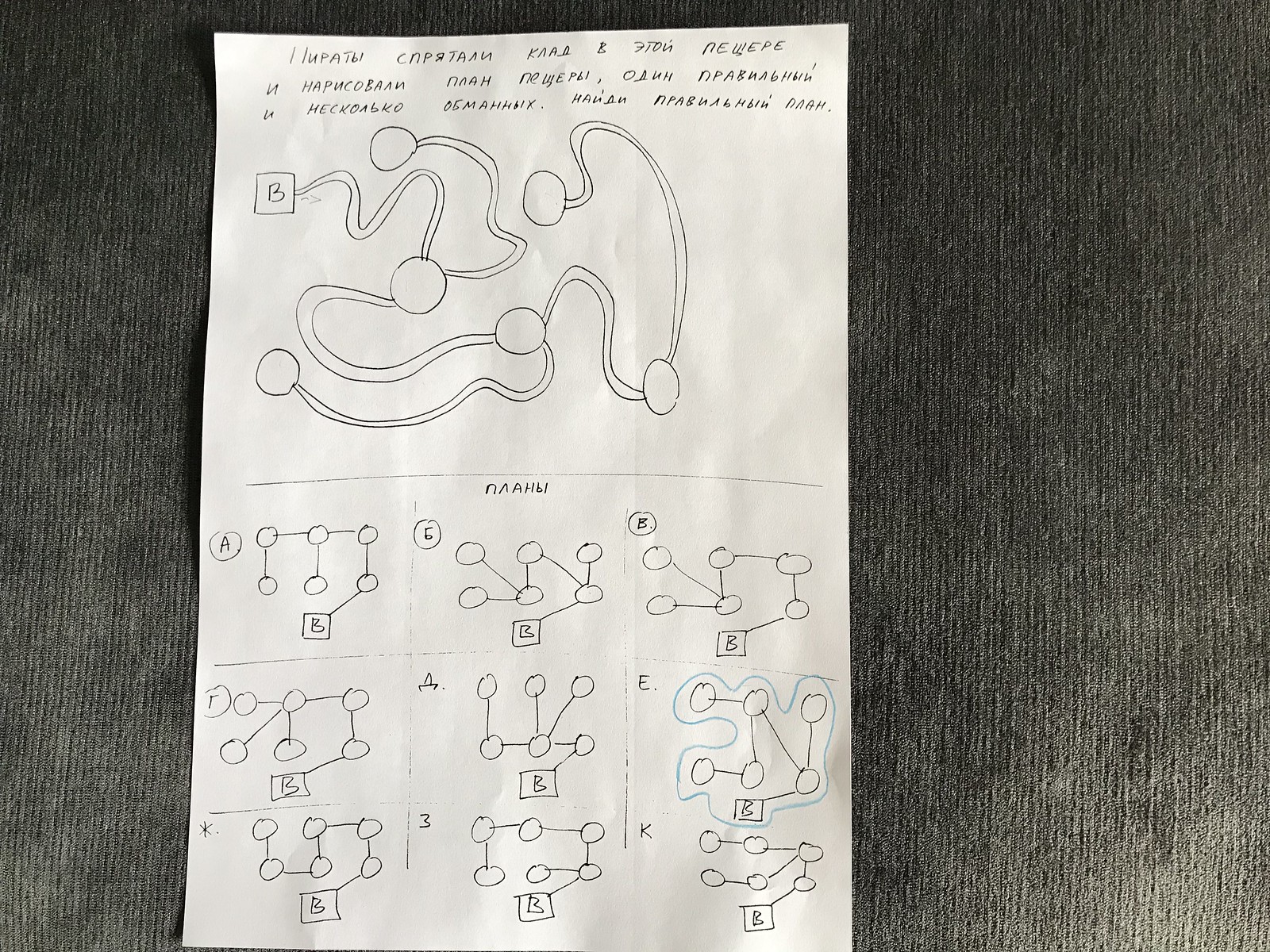The image displays a series of intricate diagrams sketched on a sheet of paper, which is placed on a gray, stitched carpet. The writing on the paper appears to be in an unfamiliar language. At the top, there are three lines of text followed by a detailed diagram. This diagram starts with the letter 'B.' From there, a curvy line spirals through a circle and then twists up and around, ending in a circle. 

Another section of the line descends, looping around to terminate in a circle with two branching paths. One path extends downward, curves back to the left, and concludes in a circle. The other path ascends, loops back down and to the right, ending in a circle as well. This pattern continues with the line curving upwards, then back to the left, and finishing in another circle.

Below this complex diagram, there is some additional text followed by a series of nine smaller diagrams. Each diagram is labeled with letters and symbols such as 'A,' 'B,' 'C,' 'A,' 'E,' 'B,' and so on, along with various configurations. These diagrams consistently show circles connected by lines, where one line segment typically ends in a square labeled 'B.' These diagrams appear to illustrate different methods of connecting circles while maintaining the same spatial orientation among them.